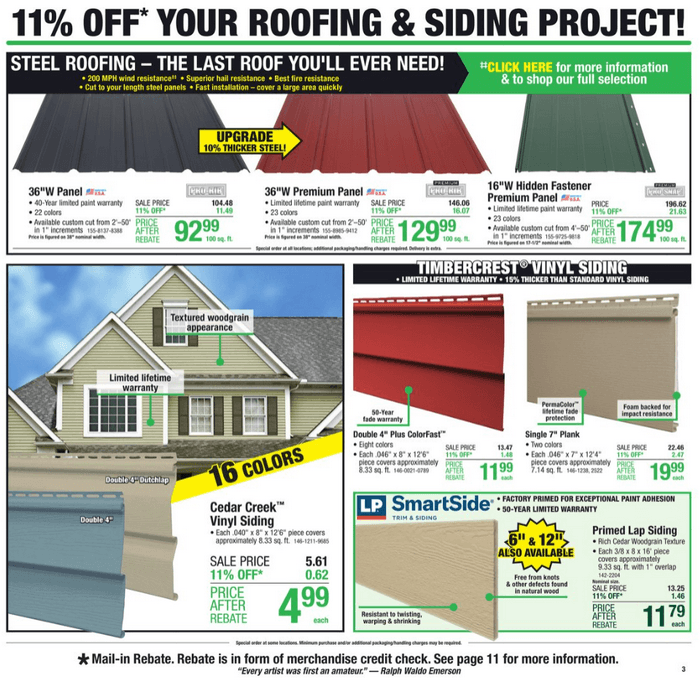This screenshot captures an advertisement for a promotional brochure, reminiscent of typical junk mail, offering a discount on roofing and siding projects. The top of the ad prominently features a bold headline declaring "11% Off," accompanied by a small asterisk providing further conditions: "11% off your roofing and siding project!" The brochure is divided into three sections for clarity:

1. **Top Banner**: This section showcases the various types of steel roofing available. It includes essential information such as pricing, estimates, dimensions, and sale prices, alongside vibrant color visuals of the different roofing options.

2. **Bottom Left**: A stock image of a house is displayed, highlighting its roof. This segment focuses on visual appeal and details additional information in a yellow banner stating "16 Colors," the price after the rebate, and the types of roofing panels available.

3. **Bottom Right**: This portion provides more detailed descriptions of each type of roofing panel. It also features an association with the company SmartSide, which offers trimming and siding solutions, accompanied by related details.

Overall, the brochure is designed to be visually engaging and informative, drawing the viewer's attention to the various offers and specifications of the roofing and siding products.